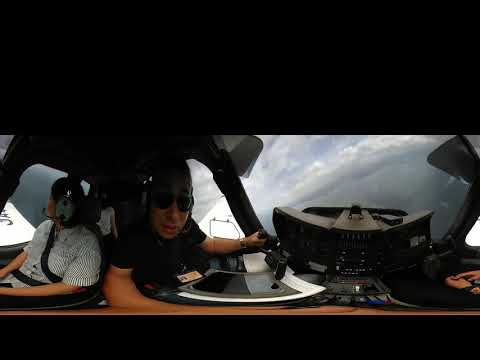In a dark, airborne setting, likely the cockpit of an airplane or helicopter, two individuals are prominently featured against a backdrop of stormy, gray-blue skies. The person on the right, wearing dark black sunglasses and a short-sleeved black shirt, holds a camera and looks directly at the viewer. He is equipped with a gray headset that includes a mouthpiece, suggesting active communication. To his left, another individual, possibly a woman, dons a striped shirt and similar gray headphones. This person faces slightly to the side, seen in profile, and is also secured with a seatbelt. The cockpit brims with numerous black controls and buttons. Through the left-side window, the wing of the aircraft is partially visible, inscribed with the letters "JA." The overall scene suggests a tense and high-altitude environment with foreboding rain clouds enveloping the aircraft.